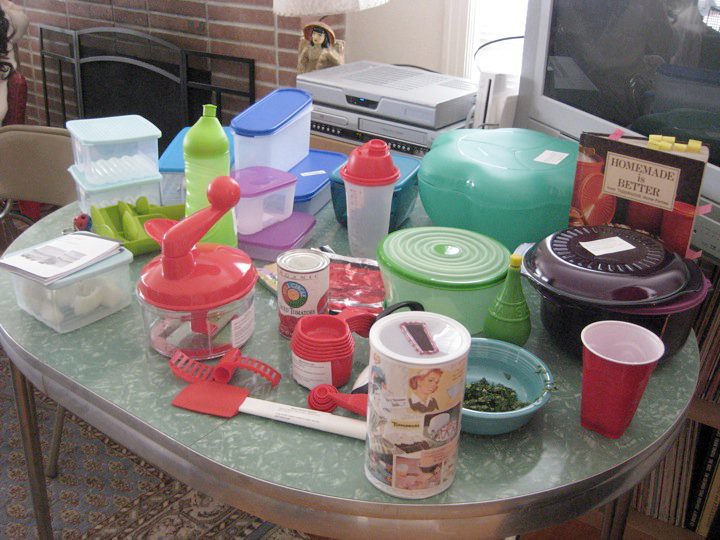This image captures a vintage dining room scene centered around a 1950s-style kitchen table. The table, featuring a light green and white patterned top encased in shiny metal edges, serves as the focal point. No chairs are present, amplifying the table's utilitarian atmosphere.

The table is cluttered with an assortment of kitchenware, predominantly Tupperware containers in various shapes and sizes, all except one sealed tight. In the foreground lies a red spatula with a white handle alongside an ice cream scoop featuring matching red accents. An open container designed for dispensing, adorned with early cartoon illustrations, catches the eye though its contents remain ambiguous.

A blue bowl appears brimming with fresh blueberries, while a single red Solo cup stands nearby. A well-read book titled "Home Made Better," marked with yellow sticky notes, hints at frequent use and culinary inspiration. Adding to the visual curiosity, a green-filled bowl, possibly containing green bananas or another mysterious ingredient, remains open.

A nearby device, used for spinning or mixing, has a clear body and a red top, further contributing to the kitchen’s eclectic mix. In the backdrop, an old VCR/DVD combination sits beneath a vintage tube television, adding a nostalgic touch to the domestic collage.